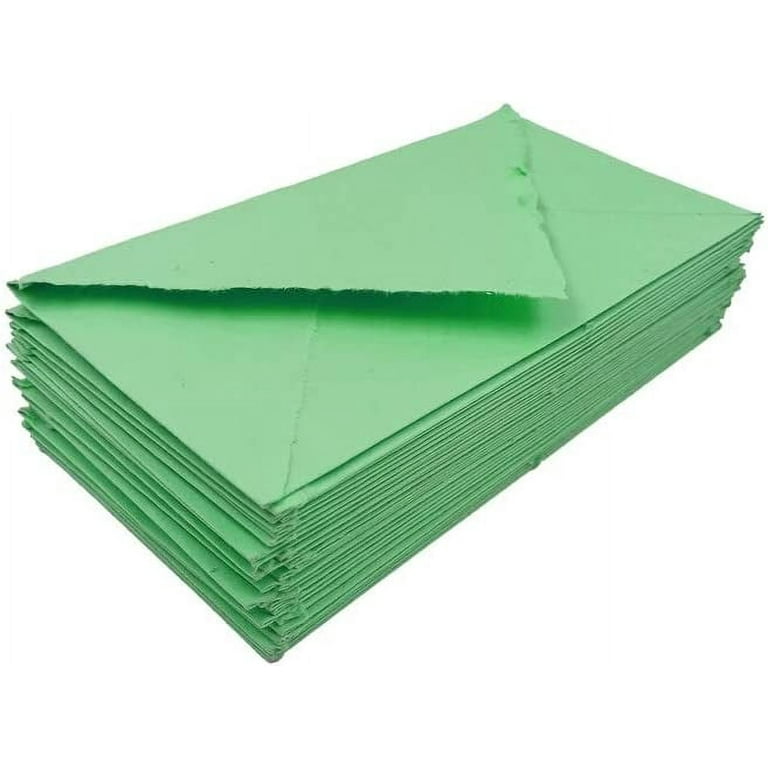The image features a stack of approximately 20 to 30 green envelopes, prominently displayed against a white background. These envelopes appear to be crafted from thick, kraft paper and have a distinct, aged look created by their deliberately torn or shredded edges. The triangular flaps, which are unsealed, point downwards and cast subtle shadows underneath due to being slightly raised. The stack is arranged at a slight angle, with some envelopes offset from left to right, adding to a casual, handmade aesthetic. The overall impression is one of artisanal quality, perhaps suitable for sending special or novelty messages.